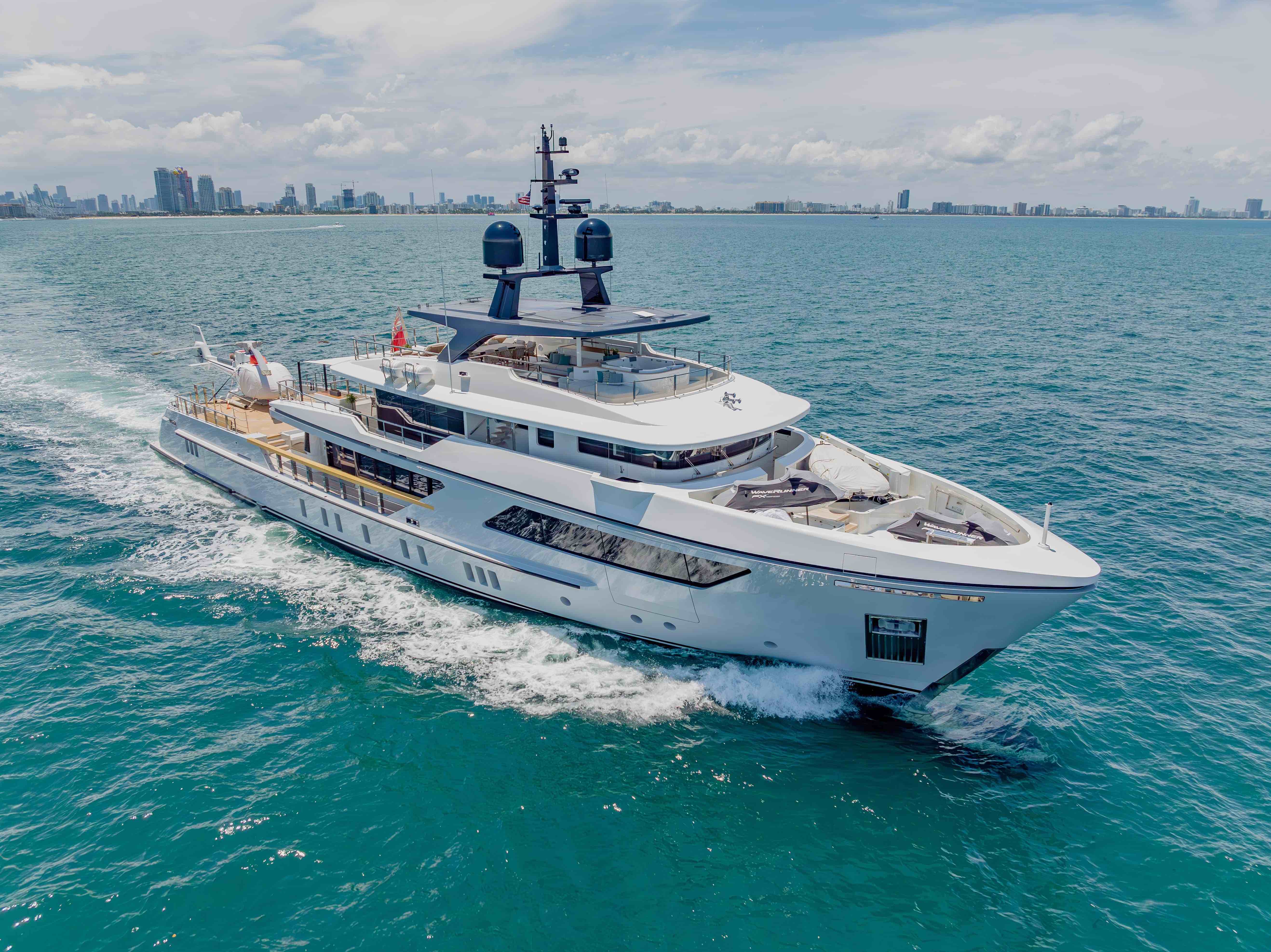A stunning photograph features a sleek, white yacht cruising through clear turquoise waters. The aft section showcases a blonde-wood deck, resembling a helipad, where a pristine white helicopter with red and blue accents is stationed. The yacht is adorned with gunmetal-colored fixtures on its upper deck and boasts expansive windows offering a glimpse inside. Above the vessel, fluffy white clouds float in a blue sky, while sunlight reflects off the yacht's white and blue accents, adding a sparkling touch. Towards the bow, a slender metal object, likely an antenna, rises up. The American flag waves at the stern, blending harmoniously with the foam trail left by the yacht's movement. In the backdrop, an impressive city skyline adds an urban contrast to this maritime scene.